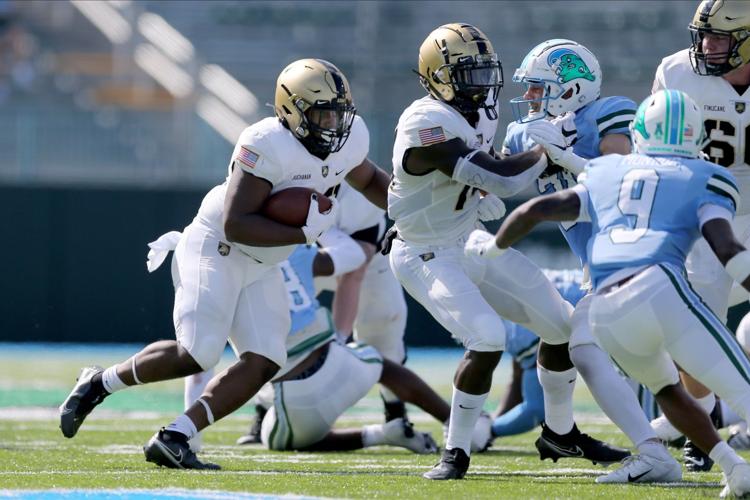In this dynamic and somewhat blurry photograph taken during a lively football game under a sunny sky, players from opposing teams are captured in mid-action on a green, turf field. The image features a mix of African-American and white players, split between two teams distinguished by their uniforms. One team dons white jerseys, white short pants, and gold helmets with black stripes, while the opposing team is clad in light blue jerseys, white pants with blue stripes, and white helmets featuring green and blue designs. Notably, one player in a white jersey, clutching the football tightly to his chest, is seen with bent knees as if running, while his teammate attempts to fend off an oncoming opponent in a blue jersey. The match appears intense, with multiple players either charging at each other or stumbling, conveying the fierce competition. A large number "9" in white letters is also visible on the back of one of the blue team members. Despite the action, the stands in the background seem empty, indicating that the focus is purely on the players' struggle on the vividly marked turf field.